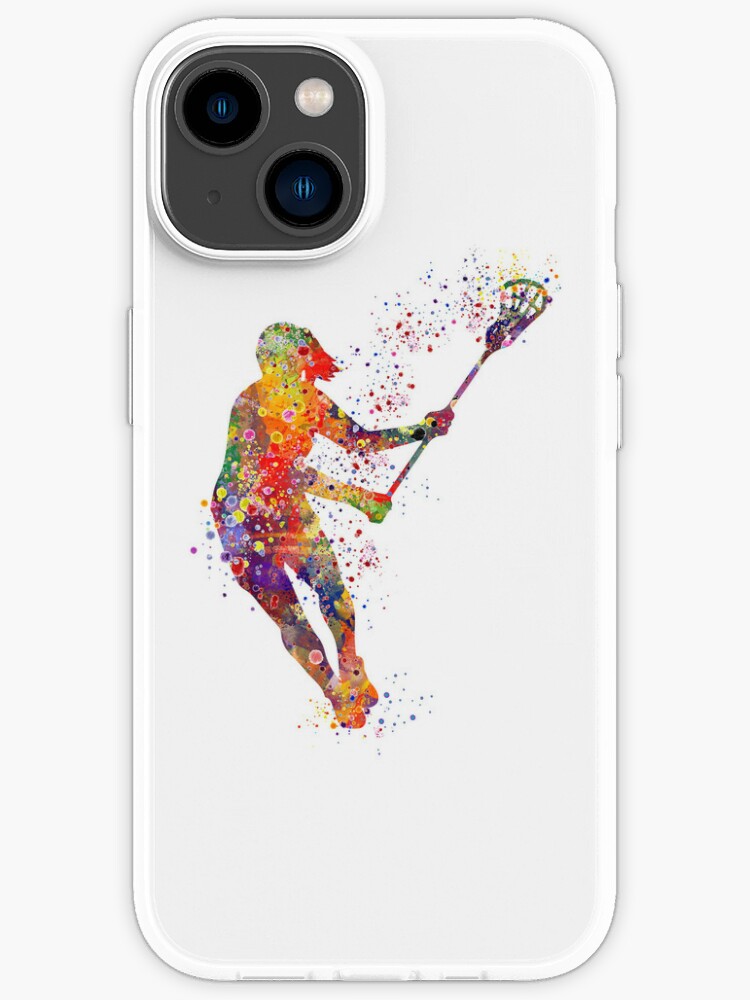This is an image of the back of a smartphone case, which could possibly be an iPhone or a Samsung model. The case is primarily white with light gray accents, including a dark gray section in the top left corner that houses the two black camera lenses and a small circular flash. 

Decorating the white case is a striking, multicolored paint-splatter silhouette of a girl in a running pose, holding a lacrosse stick with a net. The silhouette features vibrant rainbow colors, including red, yellow, green, blue, orange, and purple. The paint splatters around her and coming out of the lacrosse net create a dynamic impression of movement, as if she has just kicked up dirt during the game. Additionally, slight slivers of the phone's side buttons are visible, contributing to the overall detailed appearance of the case.